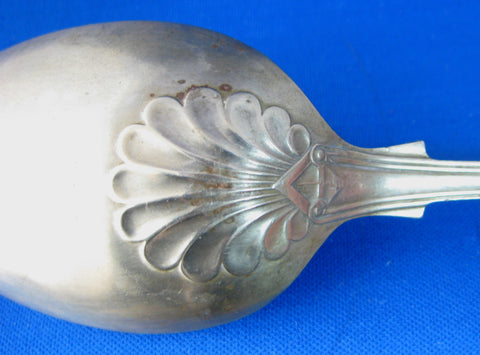This detailed color photograph in landscape orientation showcases an ornately decorated silver teaspoon, displayed upside down with its convex bottom facing the viewer. Horizontally positioned, the handle extends toward the right edge and is partially cut off, while the left tip of the spoon is also slightly cropped. The spoon features a fluted shell design that occupies about half of its bottom, aligned horizontally with the handle. Notably, there is a small triangular element where the handle meets the scallop design, and further up the handle, a fluted portion is visible as it starts to narrow. The silver surface of the spoon shows a few tarnished spots near the top part of the scalloped design. The entire spoon rests on a textured royal blue background, adding a vivid contrast to the metallic sheen. The photographic style emphasizes realism and product detailing, making the decorative elements and tarnish vividly apparent.